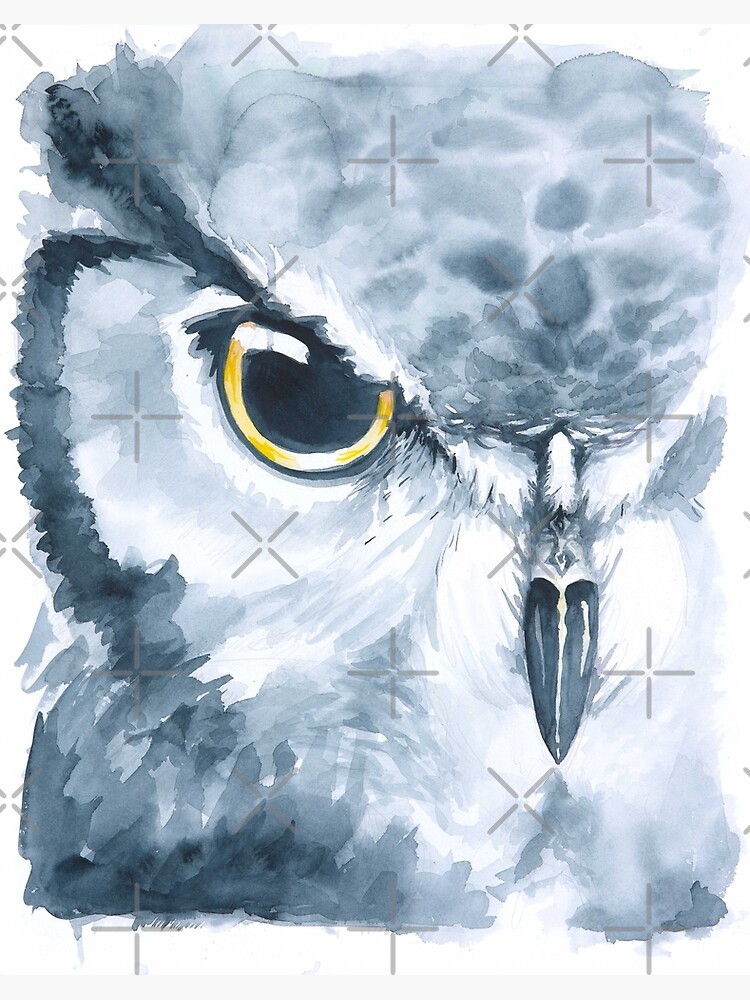This artwork is an extreme close-up watercolor painting of an owl's face, focusing solely on its right side. The owl is predominantly cyan with dark blue lining and blotches scattered throughout its features. Its striking eye is detailed with a dark blue pupil accented by a white reflective dash, surrounded by an orange and yellow iris. The dark blue beak and splashes of white add depth and texture to the image. Unique to this piece are X's and plus signs forming a graph-like pattern in the background, which overlays part of the owl's face, creating an intriguing layered effect. The image is cropped at the neck, completely excluding the left side of the owl’s face. The overall color palette includes varying shades of blue, gray, and white, enhancing the watercolor's delicate and detailed appearance.